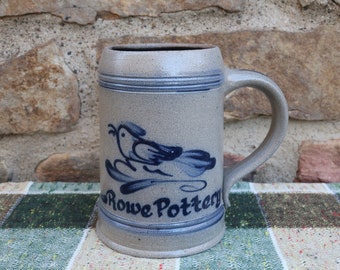In the image, there is a large, heavy-looking, grey mug situated prominently at the center of the picture, occupying about one-third of the frame. The mug features blue accents, including a blue stripe along the top and another at the bottom, with intricate blue lines encircling it. On the side of the mug, there's a detailed painting of a blue and white bird, possibly a bluebird or a blue jay, appearing as if it is singing with its mouth open while perched on something that looks like either a blue leaf or a cloud. Below the bird, the text "Rowe Pottery" is written in dark blue lettering. The mug has a large handle on the right side. It rests on a countertop characterized by green and brown vertical stripes. The background consists of a rough brick wall with visible vertical mortar lines between the bricks, displaying a brownish tone with cement-colored mortar. In the background, you can also see some brown rocks and one distinctly red rock in the bottom right corner.